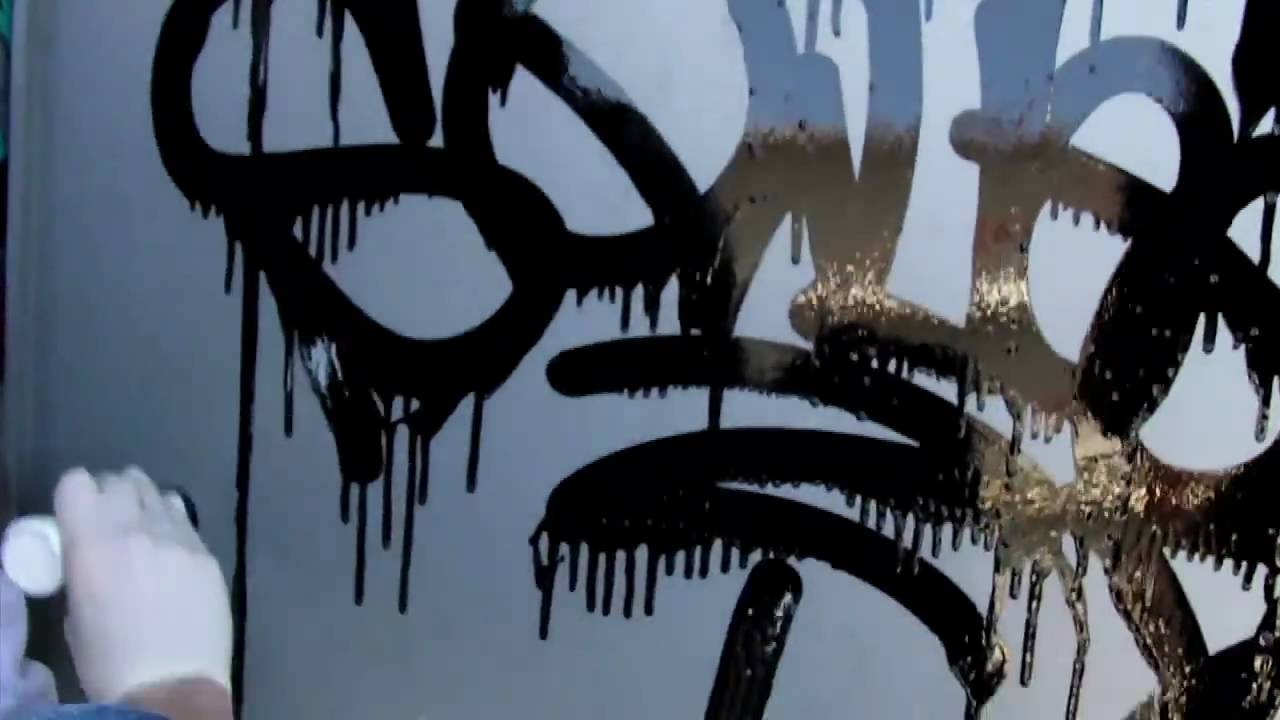This close-up photograph captures a section of a grayish-blue, potentially metal wall adorned with dripping, shiny black graffiti. The reflective nature of the black paint suggests it is still wet, with light glinting off from the right side of the image. This abstract graffiti contains various shapes, such as an 'S', a 'Z', an 'O', and a pretzel-like figure, with paint visibly running downward from these letters and shapes. In the bottom left corner, a gloved right hand wearing a latex-style glove is seen gripping a thick white marker with a black tip. The person appears to be actively painting or drawing on the wall, contributing to the chaotic yet intriguing visual of the graffiti.